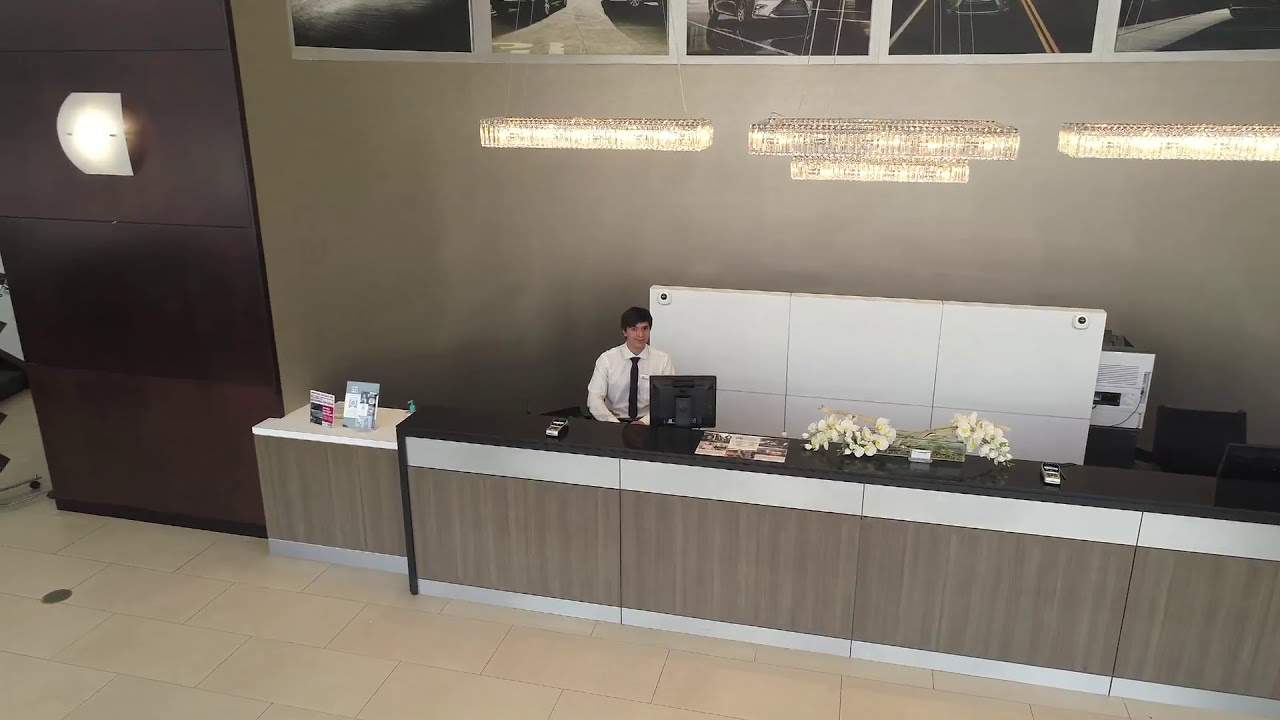The image shows a hotel reception desk viewed from an elevated angle, likely from a drone or ladder about 20 feet above. The lower portion of the picture features a white rectangular-tiled floor. The desk itself is angled diagonally, extending from the middle left section to the lower right corner of the image. It has a light wood front with gray panels and a dark stone top. 

Behind the desk, a young man in his early 20s is seated. He is wearing a white long-sleeved, button-down shirt paired with a black tie. He has black hair and sits behind a computer monitor. Arranged on the desk are a beautiful display of white orchids on a tray, a few pamphlets, and a credit card pin machine.

The background features a green wall with a whiteboard and a 3x2 white panel. High above the man, there are five windows and three lights hanging down from the ceiling, described as track lighting with rectangular crystal bars illuminating the desk area. Off to the side, a brown wooden wall is visible, enhancing the warm and inviting aesthetics of the space.